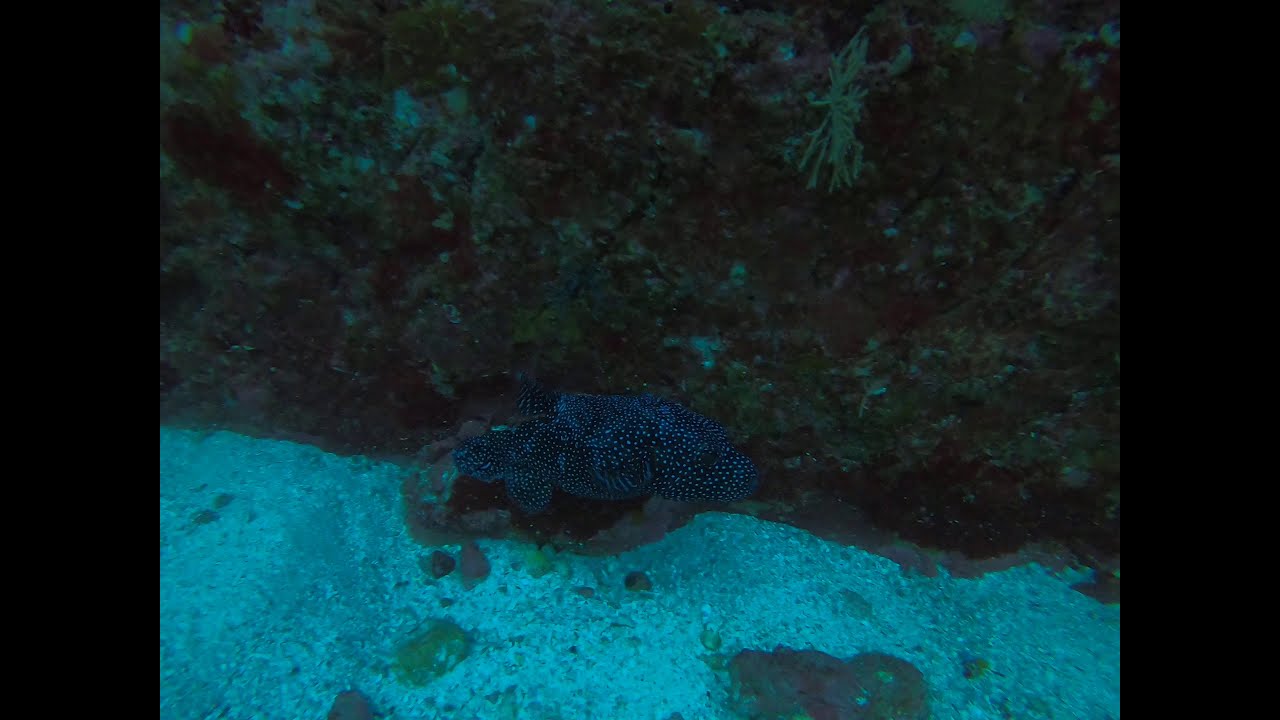This underwater image, heavily tinted in blue, captures a serene aquatic scene. Dominating the top portion of the frame is a rock wall, adorned with sediment in shades of white, tan, gray, and brown. A small green plant, likely sea grass, emerges from the rock towards the top center. The bottom section of the image transitions into a bed of white sand peppered with small yellow, tan, and brown rocks. The focal point, situated in the very center of the image, is a round, black fish adorned with white dots, its eyes gazing to the right. This detailed slice of marine life, with clear blue waters and scattered vegetation, paints a tranquil picture of an underwater ecosystem.